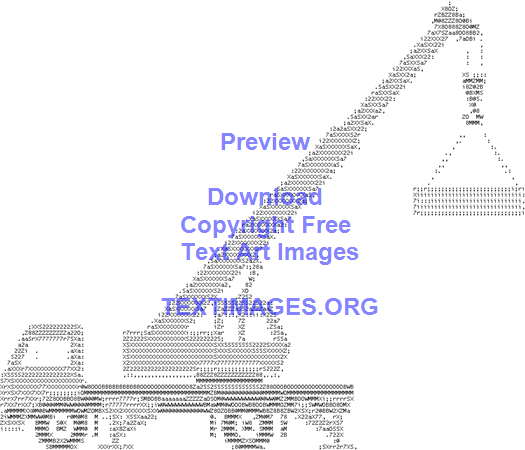This image, presented without a border, appears to be an advertisement for textimages.org, a company offering copyright-free text art images. The main graphic features a crane truck rendered entirely in light and dark grey letters and numbers, creating a dot matrix-like effect. The truck, moving from right to left, has an extended crane holding a rectangular box. Overlaid in bold, blue text is the message: "Preview Download Copyright Free Text Art Images," along with the URL "textimages.org." A light lavender watermark further identifies the image, emphasizing the crane truck's artistic composition made from textual characters.